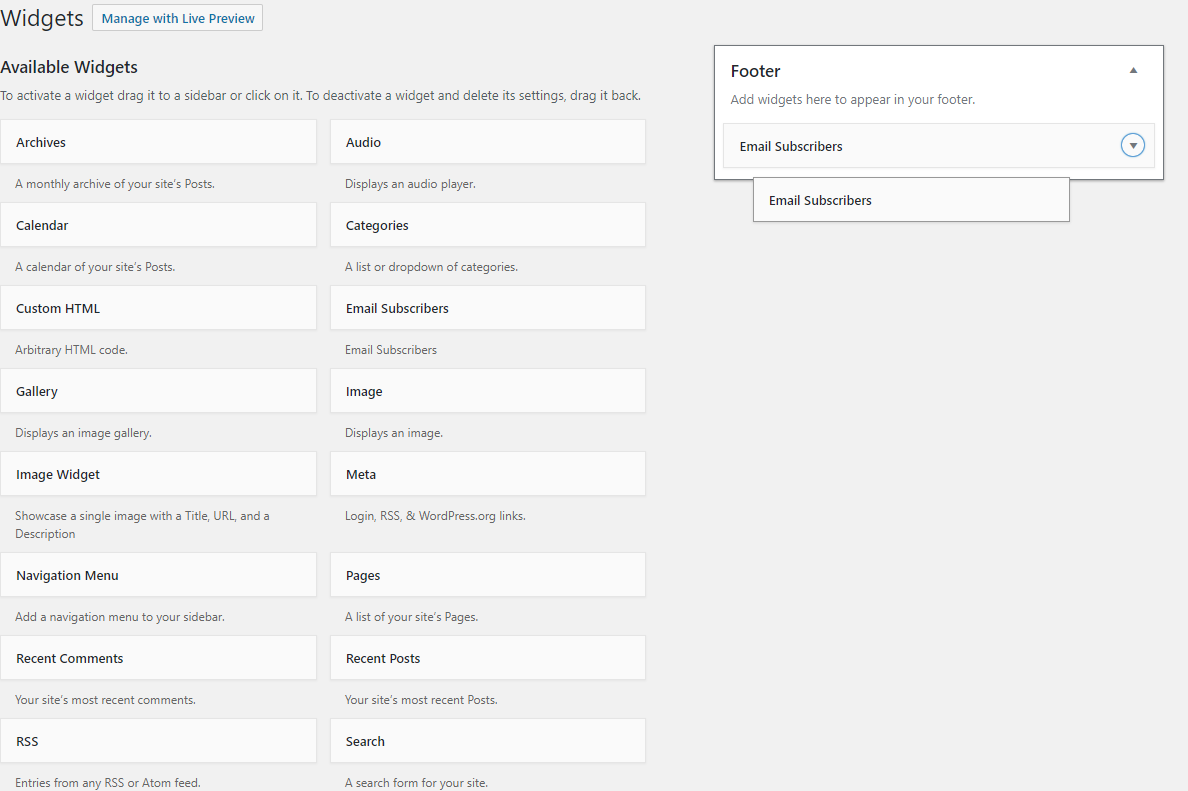This image is a landscape-oriented screenshot of a computer or laptop interface featuring a widget management screen with a gray background. At the top left, the word "Widgets" is displayed in black font. Next to it, a white text box with blue font reads "Manage with Live Preview." Below this header is the section titled "Available Widgets." Accompanying text in gray instructs users to "activate a widget, drag it to the sidebar, or click on it. To deactivate a widget and delete it, drag it back."

To the right, there's a white box labeled "Footer" in black font, with gray text underneath indicating "Add Widgets Here to appear in the footer." Above this section is a small up arrow, and below it, a prominent gray horizontal rectangle labeled "Email Subscribers," with a down arrow icon on its right side.

Within the "Available Widgets" section underneath, there are several gray rectangular boxes, each representing different widgets, including:
- Archives
- Audio
- Calendar
- Categories
- Custom HTML
- Email Subscribers
- Gallery
- Image
- Image Widget
- Meta
- Navigation Menu
- Pages
- Recent Comments
- Recent Posts
- RSS
- Search

Each widget box has a brief description beneath it. Users can add these widgets by clicking and dragging them into the designated "Footer" box in the upper right, as exemplified by the "Email Subscribers" widget already being dragged over.

The interface is clearly designed to allow users to manage and customize their website or application's widgets efficiently through a simple drag-and-drop action.